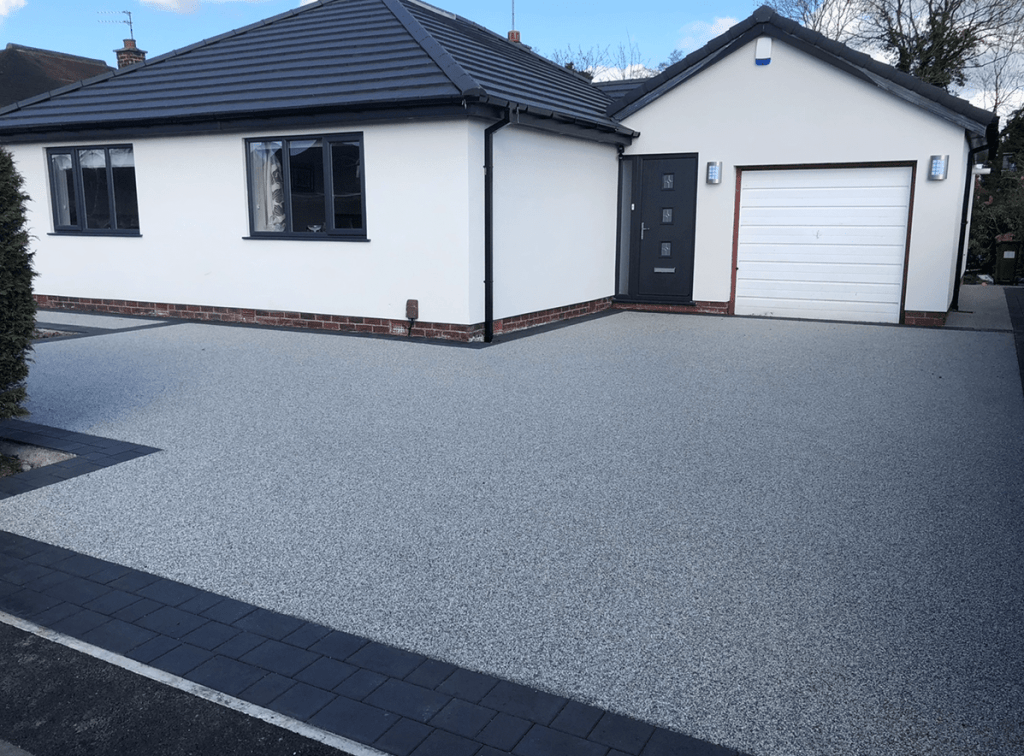The photograph depicts the front view of a remodeled, white-painted, single-story house with a simplistic design. The dark, almost navy-blue roof features two chimneys—one on the left and another towards the center. The sky above is light blue with scattered white clouds, adding a serene backdrop to the scene. The area in front of the house is paved with smooth, dotted concrete, bordered by a thin strip of pavers. Wiry trees with brown trunks and a few bushes on the left side contribute to the natural surroundings. The house's garage door is white, flanked by lights, while the front door matches the roof's greyish color. The driveway appears clean and almost new, enhancing the overall fresh and polished look of the residence.